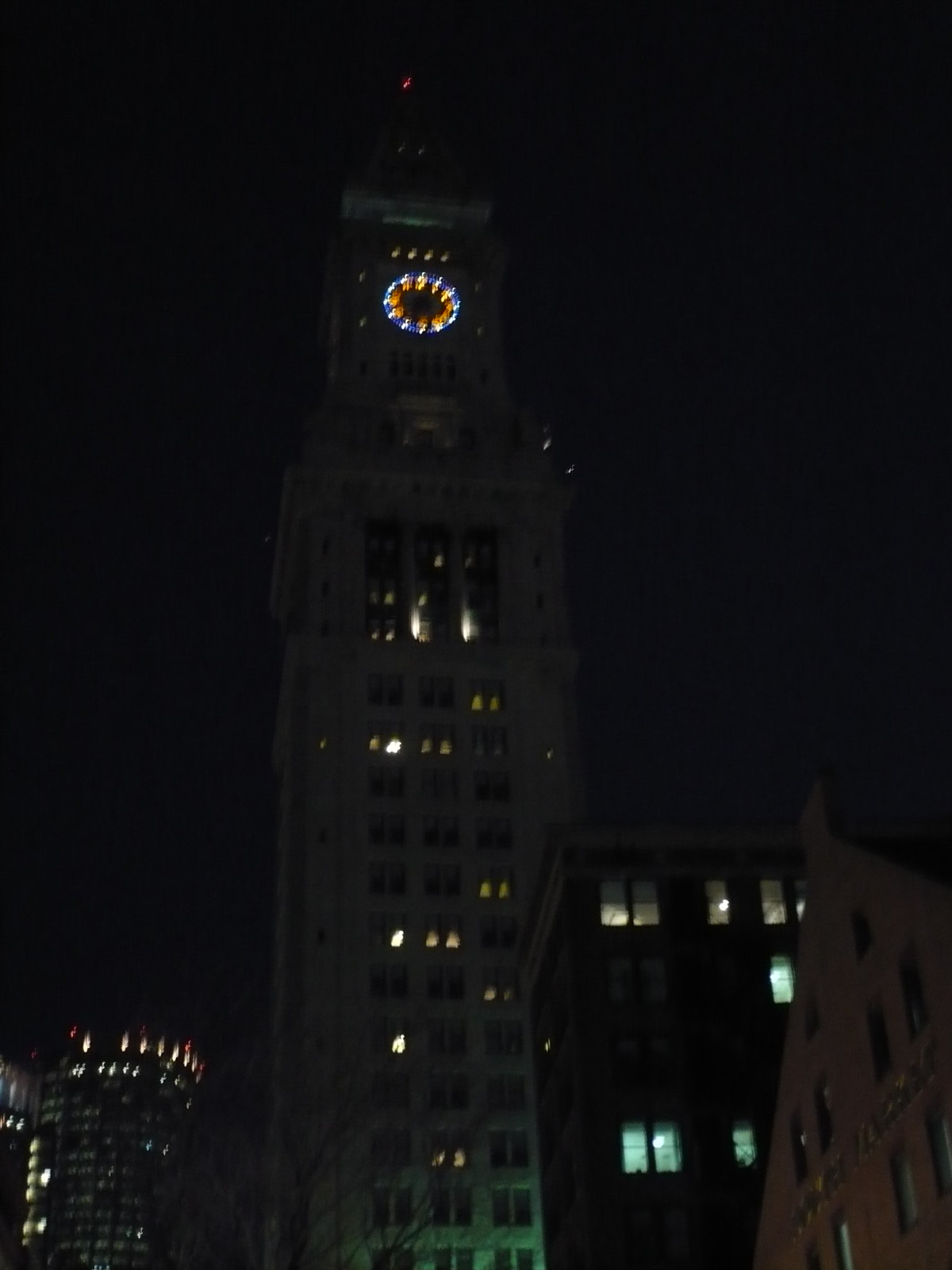This nighttime image captures a slightly blurry urban scene featuring a central skyscraper with a distinctive clock face. The sky is inky black with no visible stars or moon, save for a faint, blurred red light at the top of the tower, likely an antenna beacon. The tower, a towering concrete structure, features an illuminated clock about midway up its facade: the numbers of the clock glow a vivid orange, while the outer ring emits a striking blue hue. The majority of the tower's windows are dark, but a few are lit, contributing to the scene's overall ambiance. From the building's base, a green glow subtly rises, adding an eerie contrast to the otherwise night-shrouded buildings.

Surrounding the central skyscraper, there are several other high-rise structures. To the immediate right is what seems to be a residential building, characterized by its dark and intermittently lit windows. Further right in the foreground, another building with a triangular-shaped, peaked roof and a slightly visible inscription on its facade stands out in the night. On the left side of the frame, there's a high-rise apartment complex, equally imposing but dimly lit. A leafless tree—indicative of a possible winter setting—occupies the bottom near the base of the clock tower, its branches starkly outlined against the darkness. The blurred elements and varied illuminations of this urban landscape create a mesmeric nighttime cityscape rich in detail and atmosphere.